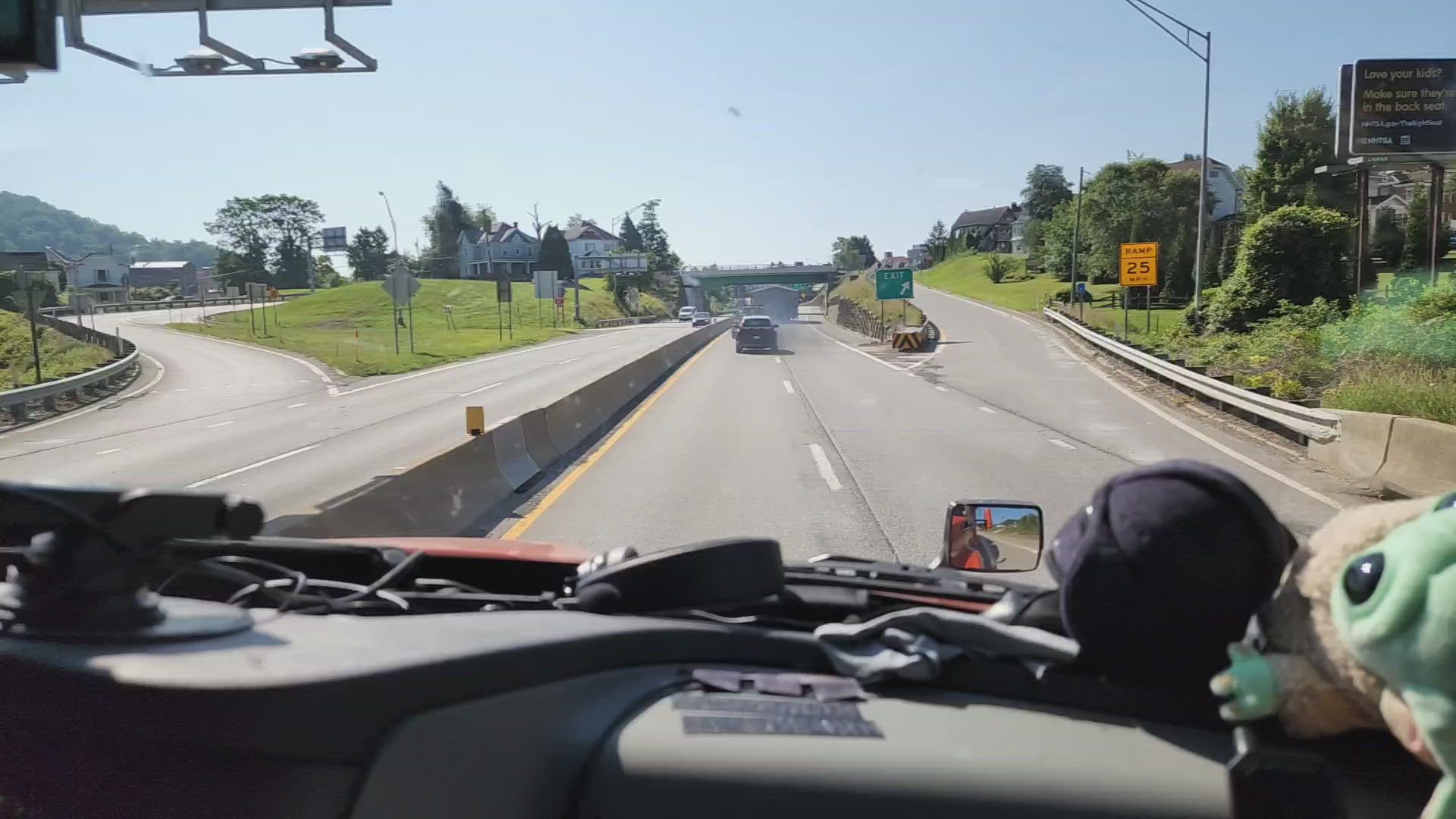The photo is taken from the passenger seat of a vehicle traveling on a two-lane highway. The dashboard is gray with a dark gray section to the left. Sitting on the dashboard are a Baby Yoda plush and a plush head of Darth Vader. In the center of the dashboard, there's a headset, and a radar detector or dash camera is mounted to the left. A small piece of the vehicle's red hood is visible. The scene outside shows an exit ramp on the left with a yellow square sign that reads "Ramp 25 miles per hour," leading up a hill. The highway is divided by a concrete barrier, with two lanes in each direction. In the distance, there's an overpass where travelers can take an exit and then turn left to cross the bridge. To the right, on a grassy, hilly area, there's a billboard with a message about child safety. A large house is visible atop a hill in the background on the left. The sky is white, indicating an overcast day.